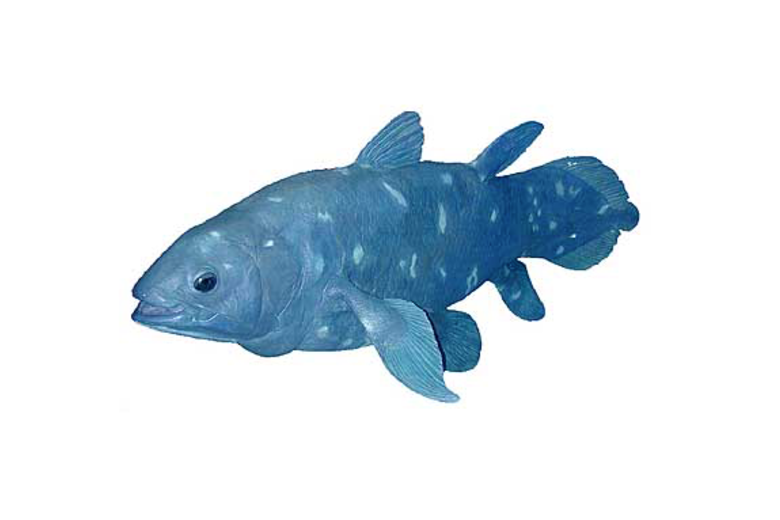The image features a blue fish set against a completely white backdrop, likely digitally enhanced to achieve this effect. Dominating the center of the frame, the fish appears either computer-generated or an older, low-quality image, with slightly fuzzy edges. The fish is of a deep, strong blue color, adorned with small, randomly placed lighter blue or nearly white specks. Shot from a side angle with its mouth slightly open, the fish showcases its left black eye and gills. It has a range of stubby fins—two top fins, multiple side fins, and a notably thick, wide tail, suggesting it might be a sea fish. The overall composition is minimalistic, featuring only the fish floating in an all-white void with no additional text or items to provide size reference.